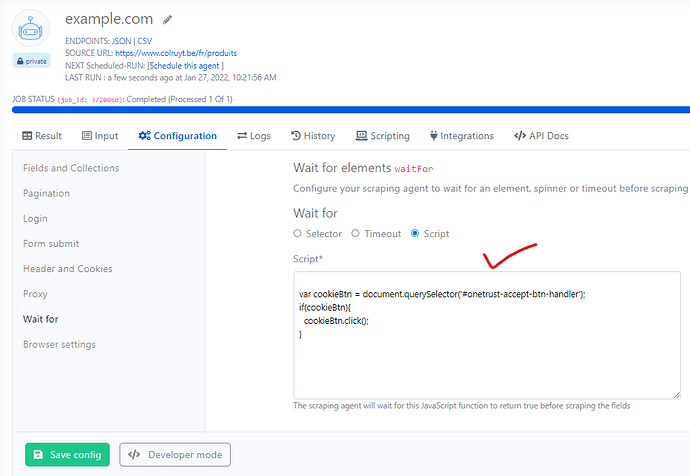In this screenshot, we are presented with a webpage tailored for configuring codes and scripts, intended for professional or expert users in this domain. The page header indicates the URL "example.com," suggesting it is a sample or demonstration page. Under the "Websites" section, several key elements are listed, including "endpoints" with options for JSON or CSV, a "source URL," the "next scheduled run," and the "last run."

Beneath these, there are various tabs and categories such as "Results," "Input," "Configuration," "Logs," "History," "Scripting," "Integrations," and "API Docs." The current view is focused on the "Configuration" tab, which contains multiple sub-options like "Fields and Collections," "Pagination," "Login," "Form Submit," "Header and Cookies," "Proxy," "Wait For," and "Browser Settings." The "Wait For" option is presently selected.

Within the "Wait For" section, a script interface is displayed, featuring fields for "selector," "timeout," and "script." The page exudes a technical and complex atmosphere, aligned with the needs of seasoned professionals who require detailed control over web scripting configurations.